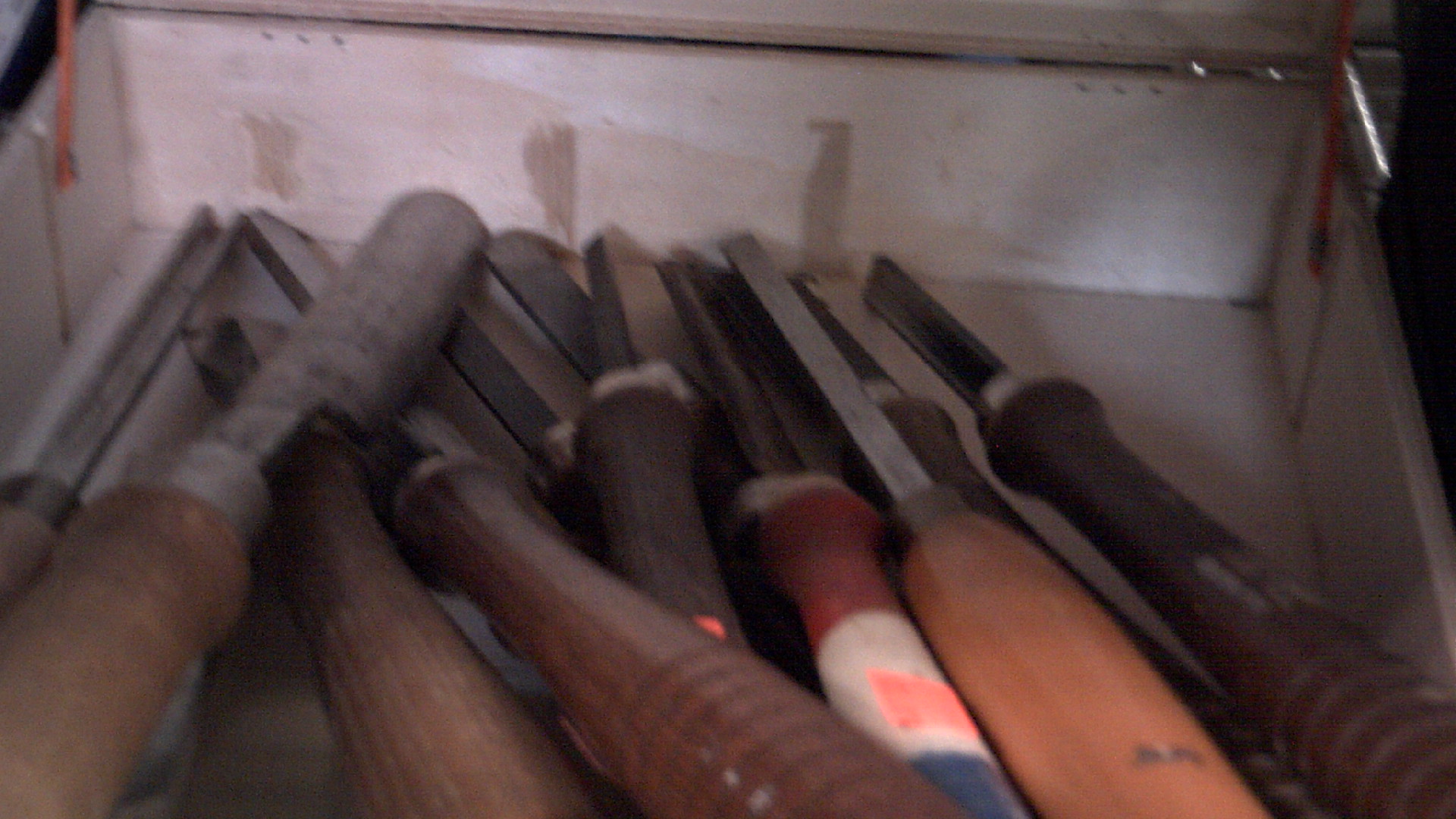This image depicts a blurry, white wooden drawer with slightly scraped surfaces. The drawer, featuring silver tips at the corners on the right-hand side, contains several metal instruments with wooden handles. The handles are primarily dark brown or light tan wood, with one distinct handle in the middle that is red, white, and blue. The metal parts of these tools vary, including straight, wide metal pieces, some resembling scrapers, and others that look more suitable for plucking objects, indicating they are not screwdrivers. Interestingly, these tools are described with terms akin to barber-like razor bases and blades. The drawer appears shallow and holds the instruments close together, which makes specific details harder to discern due to the image's blurriness.